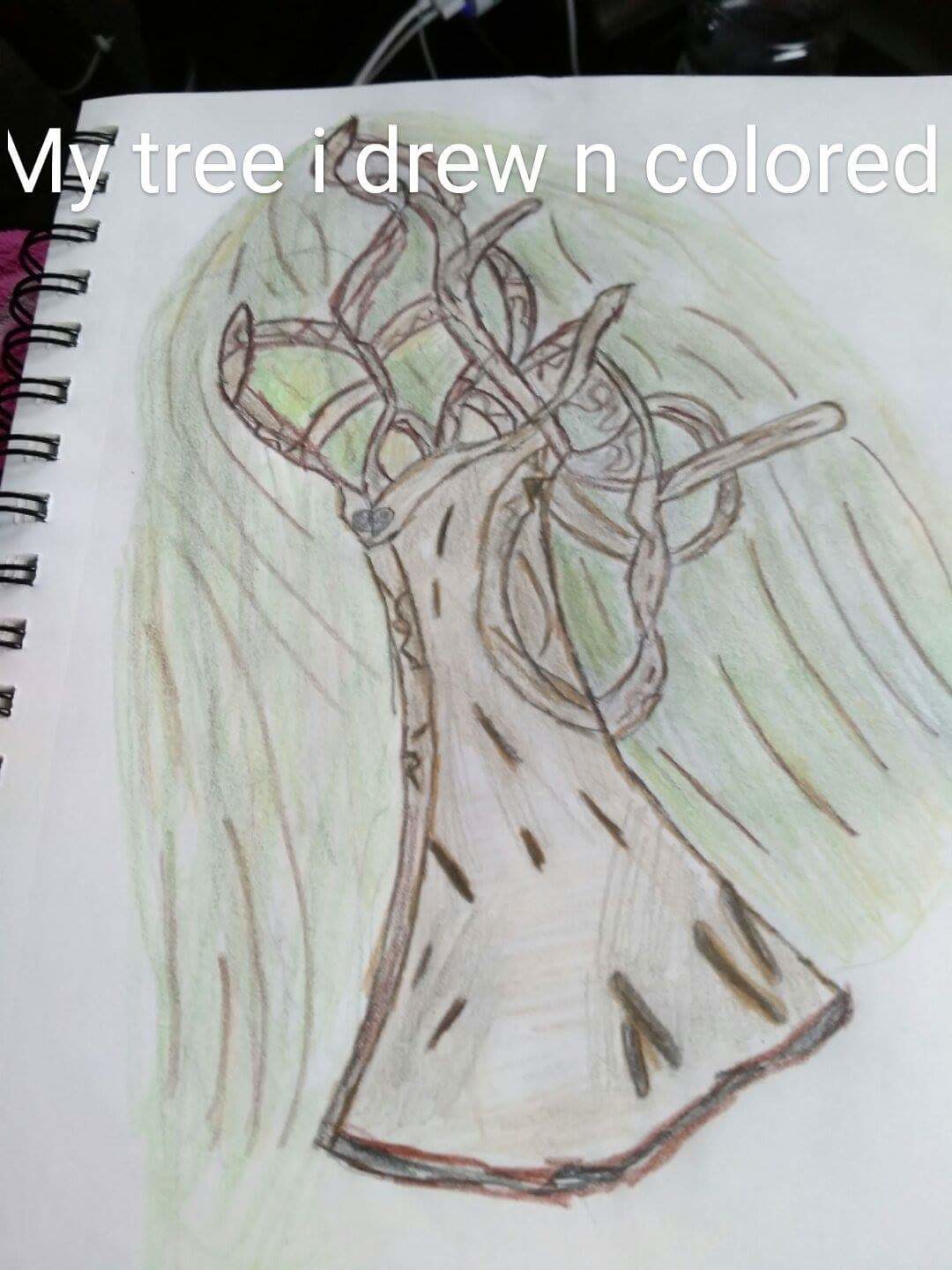In this image, there is a hand-drawn picture on a piece of white paper. The drawing appears to be an abstract representation of a tree. At the top of the page, there is text that reads, "My tree I drew and colored." The tree itself is depicted with a rough brown trunk and branches, accompanied by green coloring in the background, intended to represent foliage. The overall appearance of the tree is highly abstract and doesn't closely resemble a typical tree. Despite the artistic effort, the tree's form and structure are unconventional and may not be immediately recognizable to many viewers.